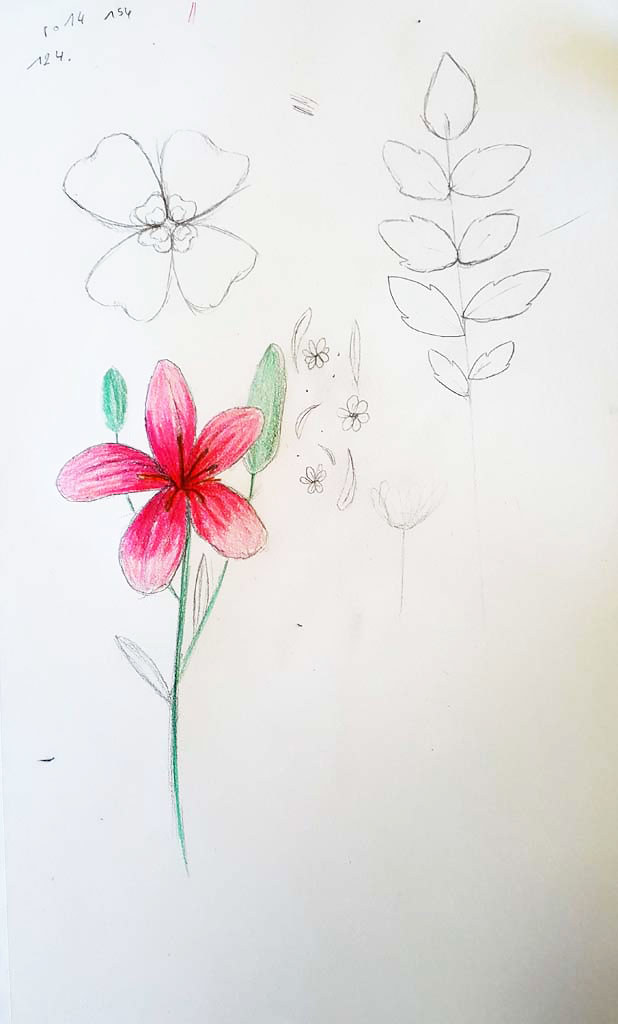The image depicts a detailed hand-drawn illustration on a white piece of paper, showcasing various plants. In the top left corner, there are some numbers inscribed, although they are somewhat difficult to discern and appear to be N54, N24, and possibly N174. This section features multiple smaller drawings, including a striking flower with four heart-shaped petals, its center rendered in pencil without any color. 

To the right of this flower, there is a depiction of a plant characterized by a stem with a leaf at the top and four symmetrical leaves on each side of the stem. On the bottom left, another flower is illustrated with a green-colored stem and several leaves that remain uncolored. This flower boasts a couple of buds and five oval-shaped petals, vividly colored in red.

The bottom right section contains additional illustrations of small flowers and leaves, all intricately drawn but lacking color. The overall composition of the drawing is a harmonious collection of flora, skillfully detailed with a blend of colored and uncolored elements.